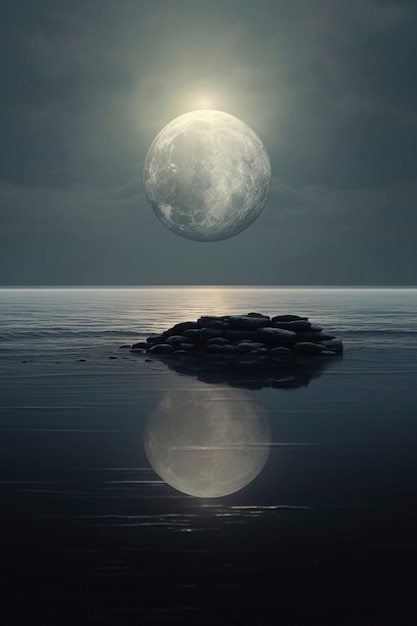This image, which appears to be a digitally-rendered artwork, depicts a surreal moonlit night over a body of water. The vertical frame is divided horizontally between the sky and the ocean. Dominating the upper half of the image is a colossal moon, with its diameter exceeding a quarter of the frame's width. The sky surrounding the moon is cloudy, showcasing various shades of gray, and there is an intense light behind the moon, possibly representing a bright star. 

The lower half features the ocean, with its surface reflecting both the moon and a small outcropping of black rocks that rises just above the water. This outcropping could be interpreted as either a series of rocks near the water's edge or a depiction of wet beach sand. The overall composition, capturing the mirrored reflections and the interplay of light and shadow, creates a tranquil yet otherworldly atmosphere, suitable for use as a phone wallpaper.